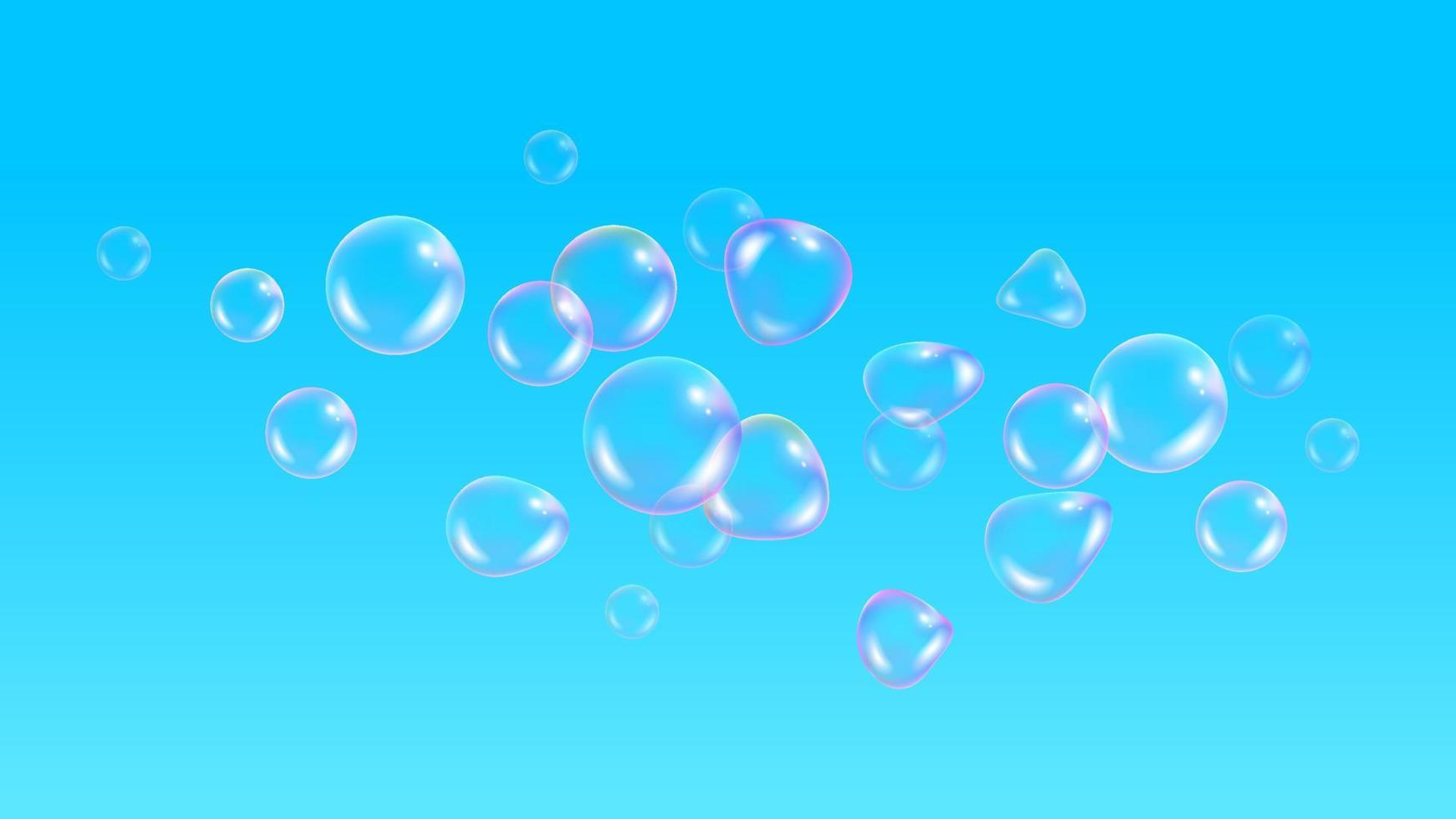In this digital artwork, a flawless, crystal-clear blue sky serves as the backdrop for a multitude of bubbles floating upwards. These bubbles, varying in size from very small to moderately large, with three notably larger ones clustered together, create a mesmerizing scene. Each bubble is meticulously detailed with a white reflection on its side and bottom, indicating a light source from the right. The bubbles display a range of iridescent colors, including purple, pink, and yellow tinges, which enhance their realistic, reflective surfaces. Scattered across the composition, some bubbles merge, while others float independently, contributing to an overall dynamic and captivating visual. The lighter blue or turquoise hue of the background, combined with the bubbles’ diverse shapes—circular, elliptical, and even some heart-shaped—adds an extra layer of depth and charm to this stunning piece, reminiscent of soap bubbles blowing in the open air.